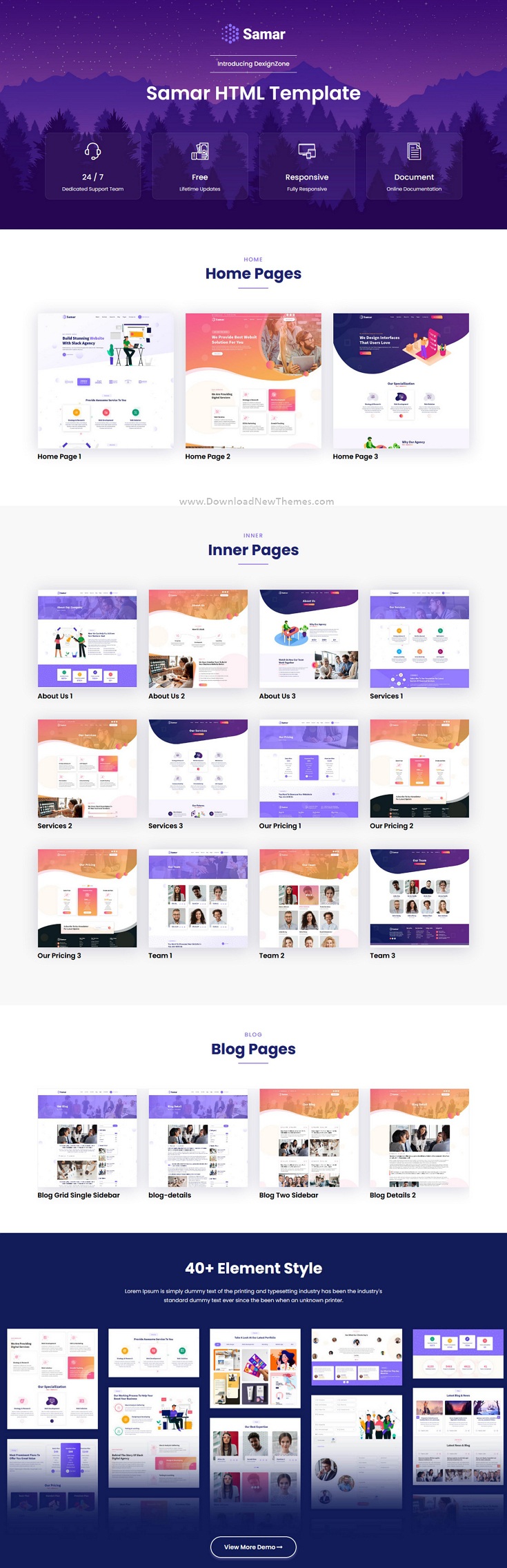This is a screenshot of a webpage displaying the Samar HTML template, albeit slightly compressed and difficult to read due to its small size and vague appearance. At the top of the page, there is a stylized graphic of a forested mountain rendered in three shades of blue, with the word "Samar" prominently displayed in the center in white font. Below this title, "Samar HTML Template" is written, followed by four clickable buttons, the labels of which are not clearly discernible.

Directly beneath these buttons is a white rectangular section labeled "Homepages," showcasing three homepage templates named "Homepage 1," "Homepage 2," and "Homepage 3." Each homepage is illustrated with a basic graphic representation of its layout.

Following the homepage section is a gray rectangular area titled "Inner Pages," featuring three rows of four template previews each. These inner page templates all share a similar, outdated aesthetic reminiscent of early 2000s web design, differentiated only by their various colored graphics.

At the bottom of the webpage, within another white rectangle, are the "Blog Pages," which offer four selections. These blog templates maintain the same design style as the inner pages and homepages, appearing visually dated and uniform in their unattractiveness.